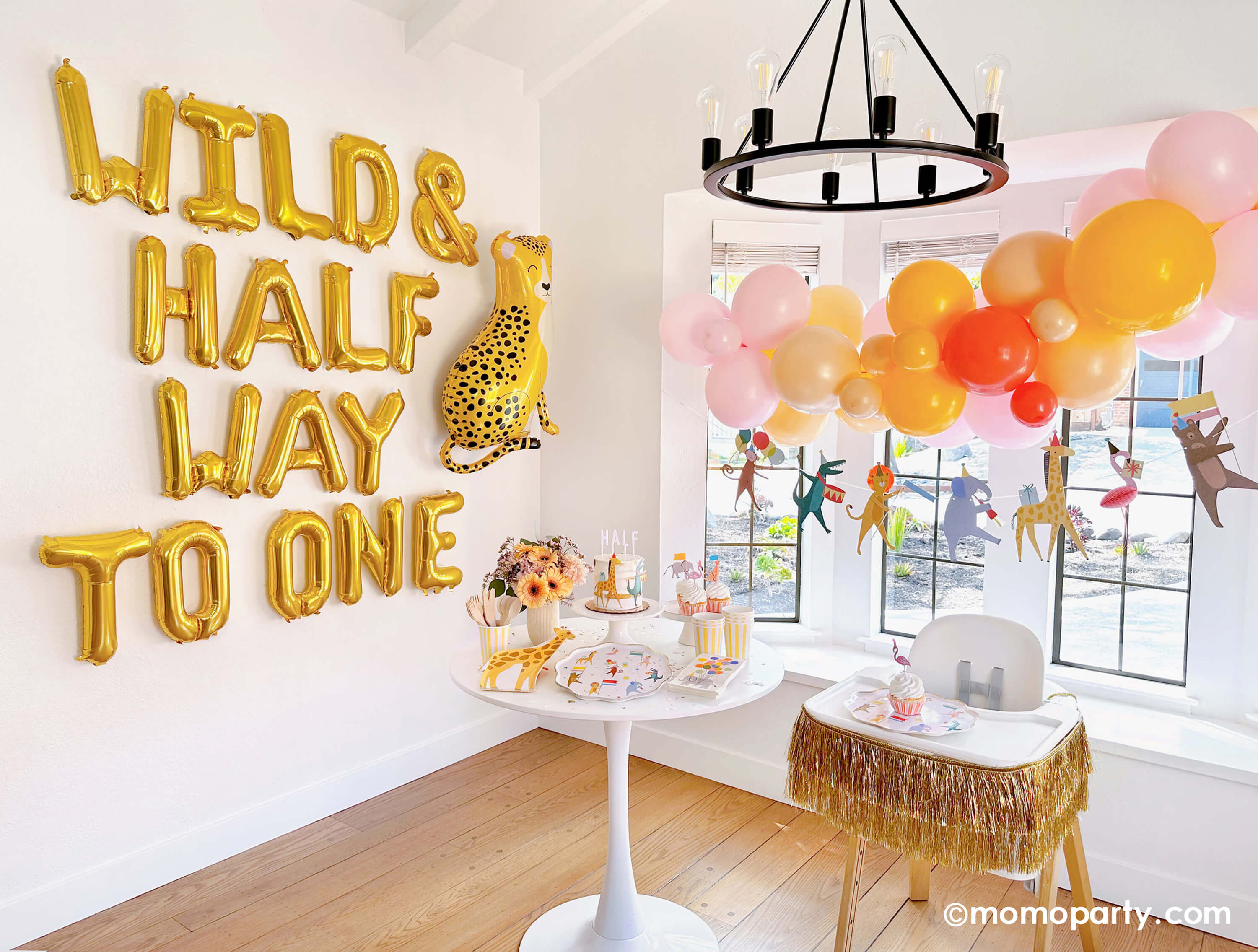A realistic photograph captures a brightly lit room in a house with horizontally oriented light brown wooden plank flooring. A large window on the right wall allows abundant sunlight, revealing a glimpse of a sunny neighborhood outside. This white-walled room appears to be the setting for a small child's birthday party, as evident from the festive decorations. 

Above, a black wrought iron chandelier with eight light bulbs adds a rustic charm to the ambience. Gold balloon letters spell out "WILD AND HALFWAY TO ONE" on the left side, accompanied by a blown-up helium cheetah balloon. Balloons in shades of pink, yellow, and red adorn the room, including a bouquet interwoven with these colors and animal cutouts dressed up for the party.

A white table is set with a variety of kid-friendly foods, cupcakes, flowers, silverware, and party napkins. Notably, a child's high chair, dressed with a stylish fringe skirt, is positioned on the right, featuring a tray with a cupcake. Additional cut-out decorations of animals like bears, giraffes, lions, elephants, and monkeys hang from the window. In the bottom right corner, the image is marked with the copyright "mom-o-party.com" in white font, attesting to its thematic design specialty.